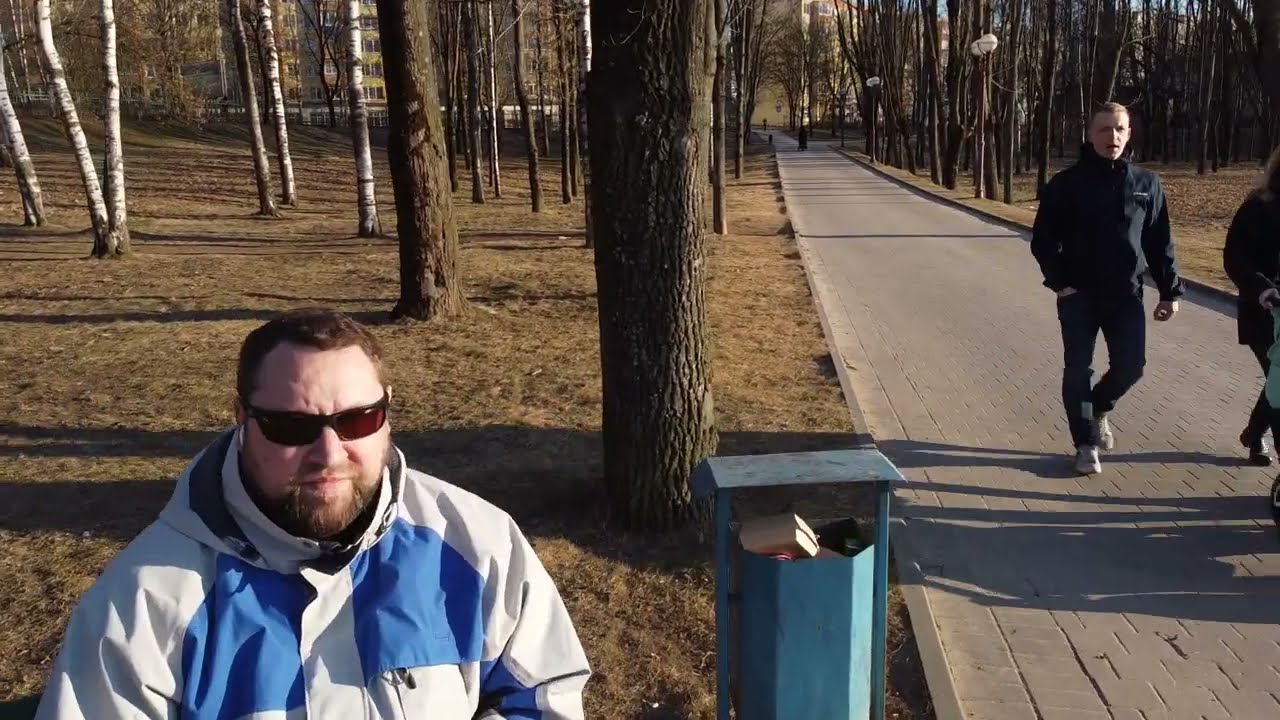This outdoor photograph features a white male with short brown hair, a brown beard, and brown sunglasses seated on a bench in the foreground. He wears a lightweight, white and blue jacket with a hood, zipped up to the collar. To his right, a teal blue metal trash can, partially overflowing with garbage, stands prominently. The scene centers around a white brick walkway, where two additional figures walk: a man dressed in black, with short hair, wearing white tennis shoes, and a woman, partially visible, pushing a stroller. The background includes numerous trees, mostly leafless, and dead-looking grass, suggesting a colder season. Additionally, the walkway is lined with lampposts featuring white globe lights. In the distance, buildings can be seen, completing the park-like setting.